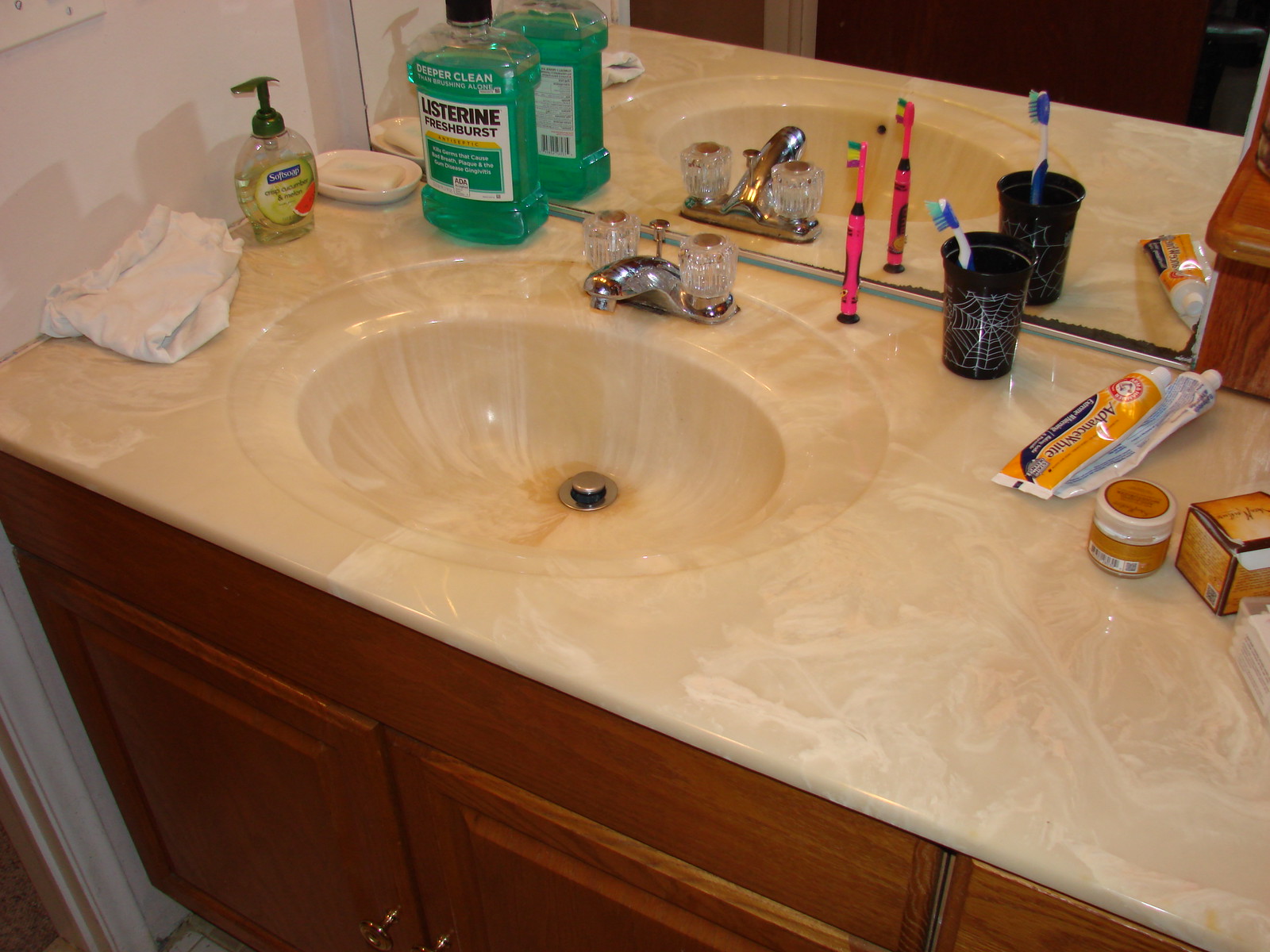This image depicts a bathroom sink area with meticulous detail. The sink is set in a white countertop, featuring an array of personal hygiene items. At the front, two cupboard doors provide storage underneath the sink. The sink itself includes a bowl with two taps—one for hot water and one for cold. A plunger is present for controlling the water level in the bowl. Above the sink is a clean, reflective mirror.

On the far left of the countertop lies a cloth or rag. Directly behind the cloth sits a clear soap dispenser filled with yellow soap. Adjacent to the soap dispenser is a soap tray holding a bar of solid soap. Next to the soap tray stands a bottle of Listerine Fresh Mint mouthwash in its distinctive green color.

Toward the center of the countertop, near the cold-water tap, there is a pink Crayola-style toothbrush. Beside it, a black cup featuring a spiderweb design holds a blue toothbrush. An orange tube of Arm & Hammer toothpaste lies next to the cup. Another unidentified toothpaste tube is lying upside-down under a tooth.

To the right of the toothpaste tubes is a small tub of cream. Adjacent to the cream is an orange box, which appears to be a container for an unspecified item. In the corner of the countertop, a small clear plastic container is visible, filled with cotton swabs. The arrangement of items suggests a well-used and functional bathroom sink area.